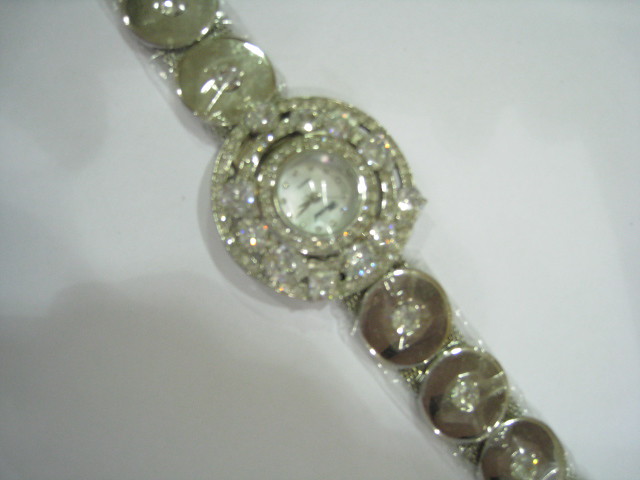The photograph captures an ornate, close-up view of a luxurious watch, meticulously designed with intricate jewelry elements. The watch face is small, circular, and features a pearlescent off-white background adorned with tiny jewel-like numbers. The golden watch hands stand delicately against this sophisticated backdrop. Encircling the watch face are concentric rings of variously sized diamonds. The innermost band is narrow, followed by a layer of larger, more spherical diamonds with prominent, faceted tops, reminiscent of engagement ring diamonds. Another narrow band of diamonds completes the circumference, adding to the elaborate detail. The watch band appears metallic, styled with circular discs that house faceted gems in their centers, creating a button-like appearance along the strap. The overall presentation suggests it may be on display in a jewelry store, laid flat on a plain white background. A shadow on the left hints at the photographer's presence, and slight blurriness around the central diamonds indicates a rushed, very close-up capture. The watch is oriented in a north-west direction, adding to its elegant positioning.